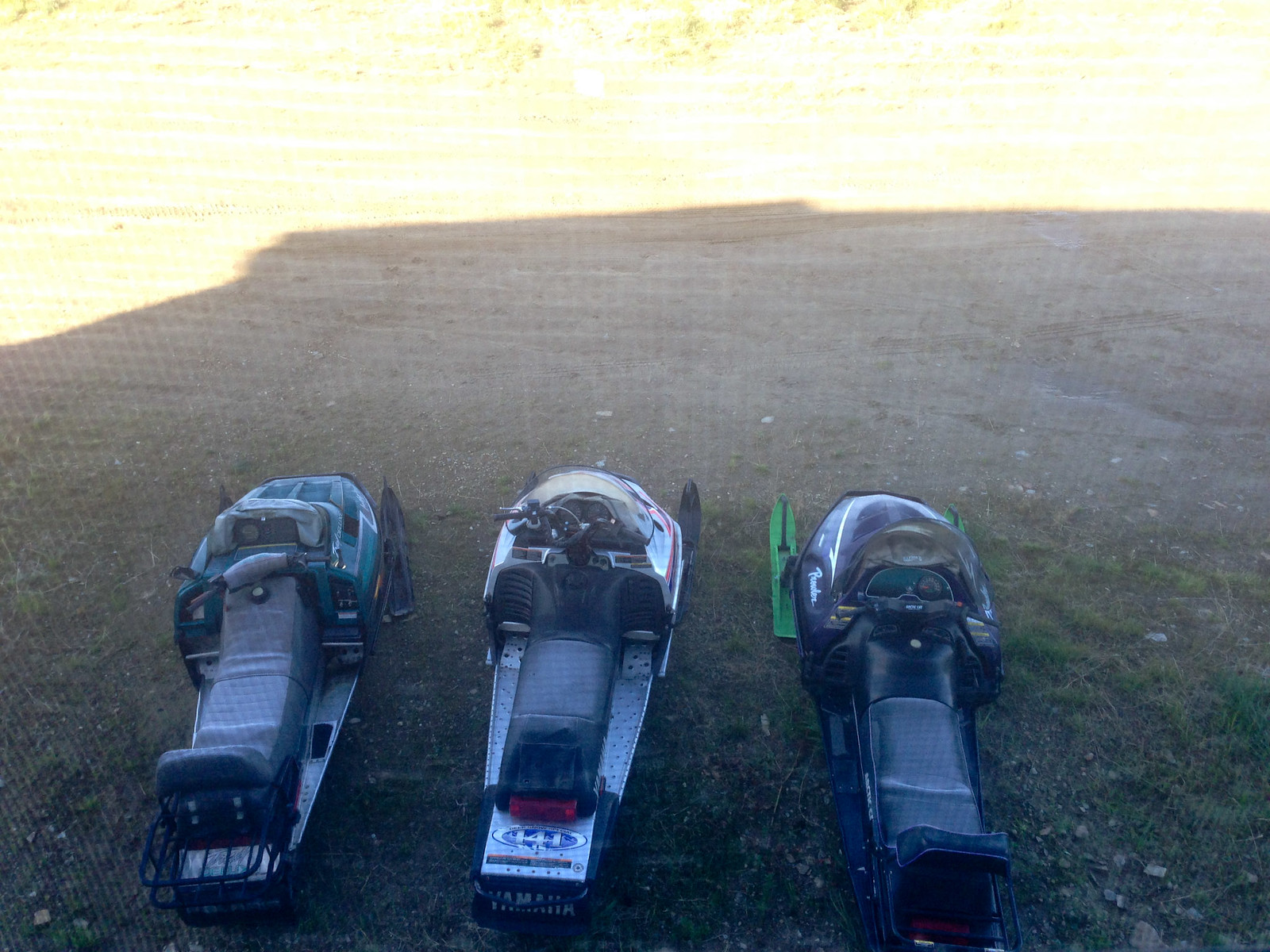In this horizontal rectangular photograph, three snowmobiles are lined up horizontally on bare ground, with their windscreens facing away from the camera. The snowmobile in the middle prominently features the Yamaha brand on its back, and has a silver, gray, and black color scheme, with black skis. On its right, the snowmobile is black with distinctive green skis, while the one on the left appears to be dark green and gray with dark-colored skis. The machines are parked on a stretch of mostly brown dirt, with sparse patches of green grass and small stones. The entire lower half of the image, where the snowmobiles are located, is enveloped in shadow, while the top part of the image is much brighter, tinged with a golden hue, likely from sunlight. The detailed composition reveals the seats, handlebars, and skis of each snowmobile clearly.